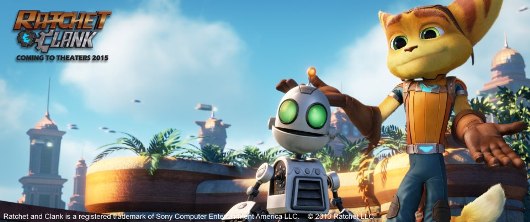The image is a horizontally-oriented poster, likely promoting either a movie or a video game titled "Ratchet & Clank". In the top left corner, the title "Ratchet & Clank" is prominently displayed. On the right side of the poster are the main characters: Ratchet, resembling a fox with yellowish-tan fur, adorned with head stripes and large ears. He is dressed in blue jeans and brown gloves. Beside Ratchet stands Clank, a silver-grey robot with striking green eyes. The background showcases a serene scene with planters containing ferns or short palm trees, set against a backdrop of white buildings and a blue sky dotted with clouds. At the bottom of the image, beginning from the bottom left corner, the text reads: "Ratchet & Clank is a registered trademark of SORNY Computer Entertainment America, LLC." This detailed setting and character design help capture the essence of the "Ratchet & Clank" franchise.